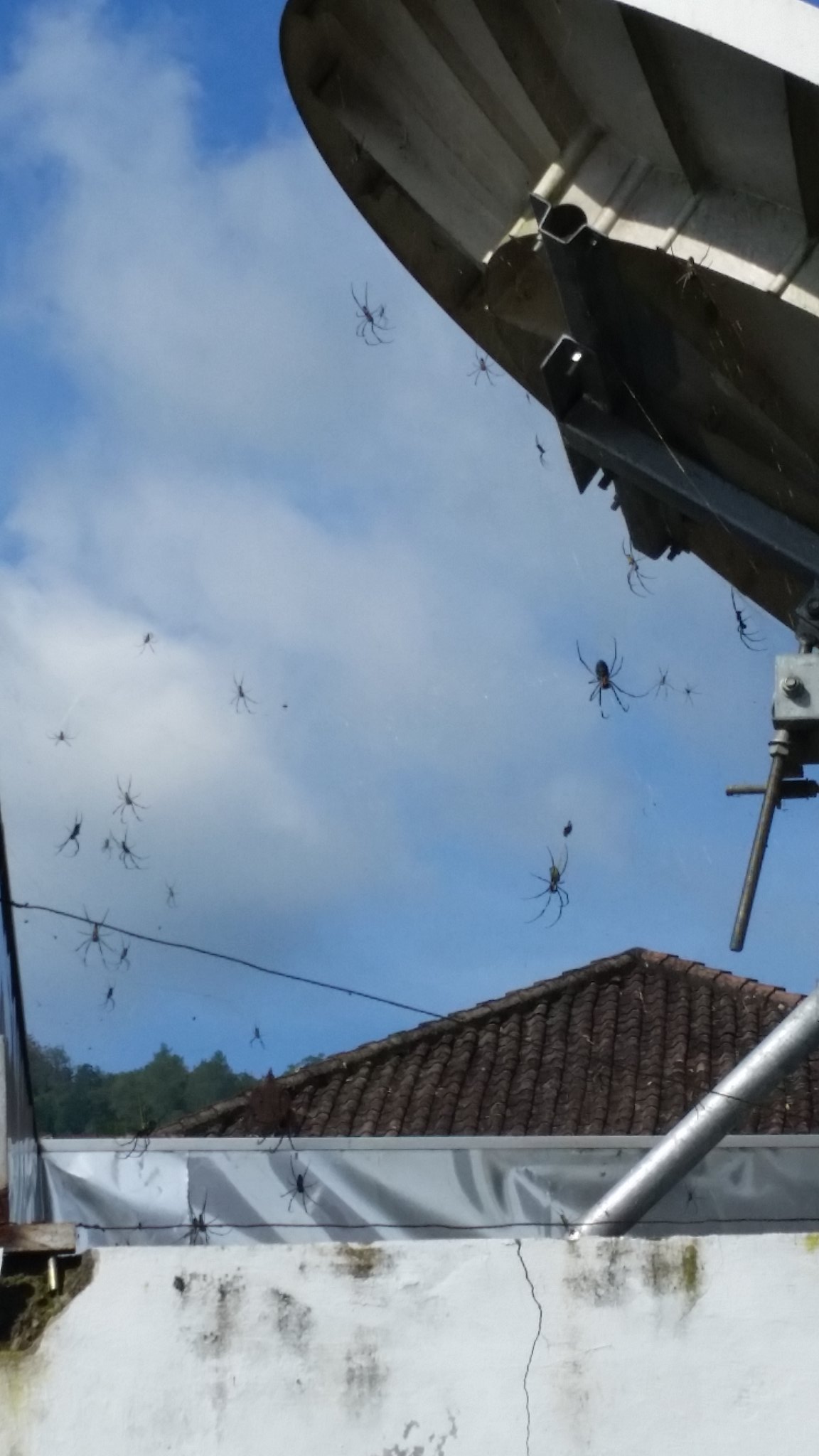This daytime outdoor color photograph captures a strikingly surreal scene set against a backdrop of clear blue skies with sporadic puffy clouds. The vantage point suggests it’s taken from a neighbor’s perspective, peering at a tiled roof crowned with what appears to be a satellite dish. The dish is mounted on a metal brace connected to the roof, and beneath it, either trailing from the structure itself or from an invisible web, dangle an impressive number of spiders. The photo shows at least twenty to forty spiders of varying sizes seemingly suspended in mid-air, giving the eerie illusion of them floating. Some of the spiders have already landed on the ledge of the roof. Adding to the unique and unsettling quality of the image, on the horizon beyond the rooftops, trees are visible, grounding the setting in a suburban neighborhood. It's a detailed, almost cinematic depiction that feels both ordinary and otherworldly.